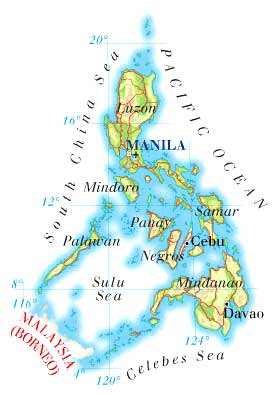This is a detailed map of the South China Sea and the Pacific Ocean on a white background. The central focus of the map includes the islands of Manila, Cebu, Palawan, Samar, Luzon, and Mindanao, all outlined with a blue drop shadow. Additional labeled areas include Mindoro, Panay, Negros, and Davao. The Sulu Sea and Celebes Sea are marked towards the lower sections of the map. In the bottom left corner, "Malaysia (Borneo)" is prominently displayed in red text, while the words "120 degrees" appear in blue text at the bottom. The bottom right corner features the label "Sulu Sea" in black text, with "124 degrees" also noted in blue just above it. The left side of the map is labeled "South China Sea," and "Pacific Ocean" is indicated on the right side.